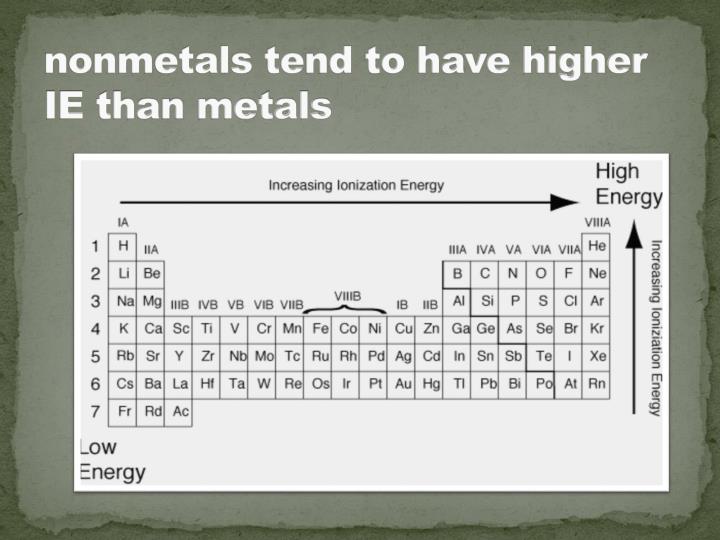The image features a detailed, color depiction of the periodic table of elements, set against a gray background with a dark gray frame. Bold white text at the top asserts that "Non-metals tend to have higher IE than metals," where "IE" stands for ionization energy. Centrally positioned is a rectangular chart resembling the periodic table, arranged into rows and columns with each cell containing element symbols. In the chart's upper right corner, black text labels "High energy," while the bottom left corner indicates "Low energy." There are two arrows: one horizontal, labeled "Increasing ionization energy," and another vertical arrow pointing upwards, also labeled "Increasing ionization energy." These arrows illustrate that ionization energy increases as you move up and to the right on the periodic table. The background texture mimics torn white paper applied to a concrete wall, adding a unique aesthetic to the scientific illustration.